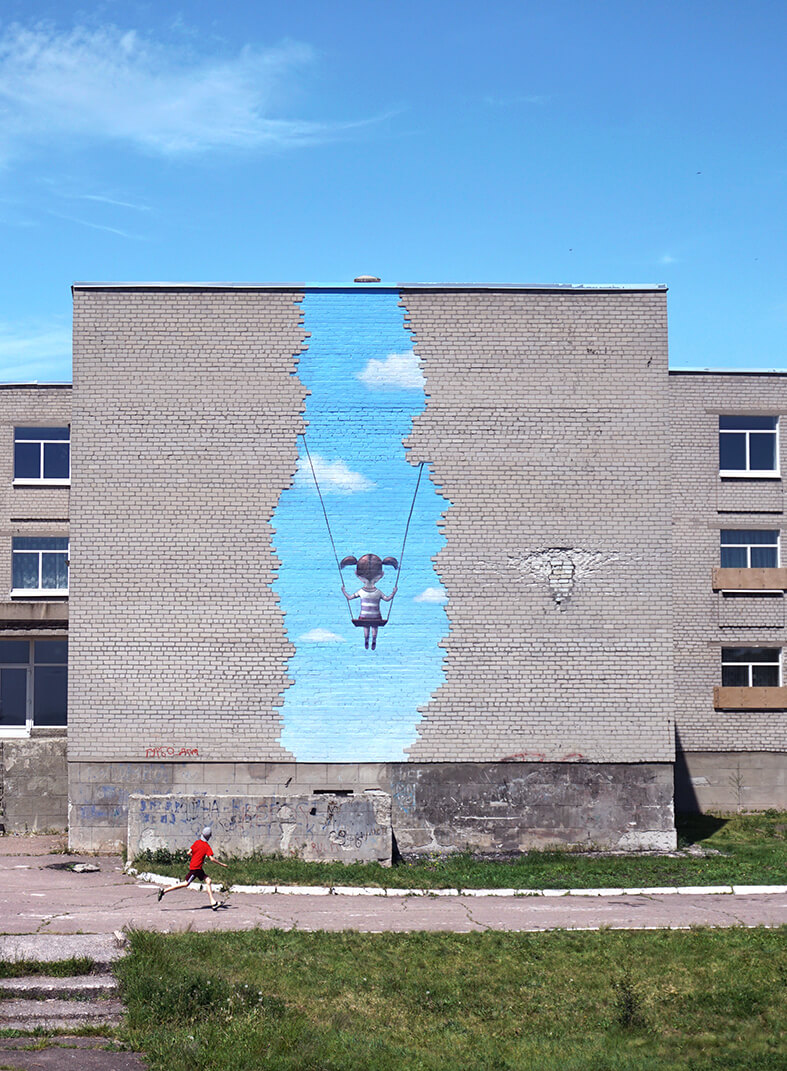This photograph captures a vivid scene featuring a large, multi-story gray brick wall adorned with a striking mural at its center. The mural, beautifully aligned with the real sky above, depicts a cartoon-like image of a girl swinging from two brick sections flanking her sides. This creative artwork creates the illusion that she is actually swinging against the backdrop of a blue sky with white clouds, seamlessly blending into the surrounding environment. Below the mural, an old, gray apartment building stands in a state of disrepair, with wooden boards covering some of its windows, further emphasizing the mural’s uplifting impact. In the foreground, a boy dressed in a red shirt, black shorts, and a backwards hat runs down a worn sidewalk, glancing up at the captivating artwork above. The surrounding grassy area and aged steps add to the contrast between the dreary building and the vibrant, hopeful message conveyed by the mural.